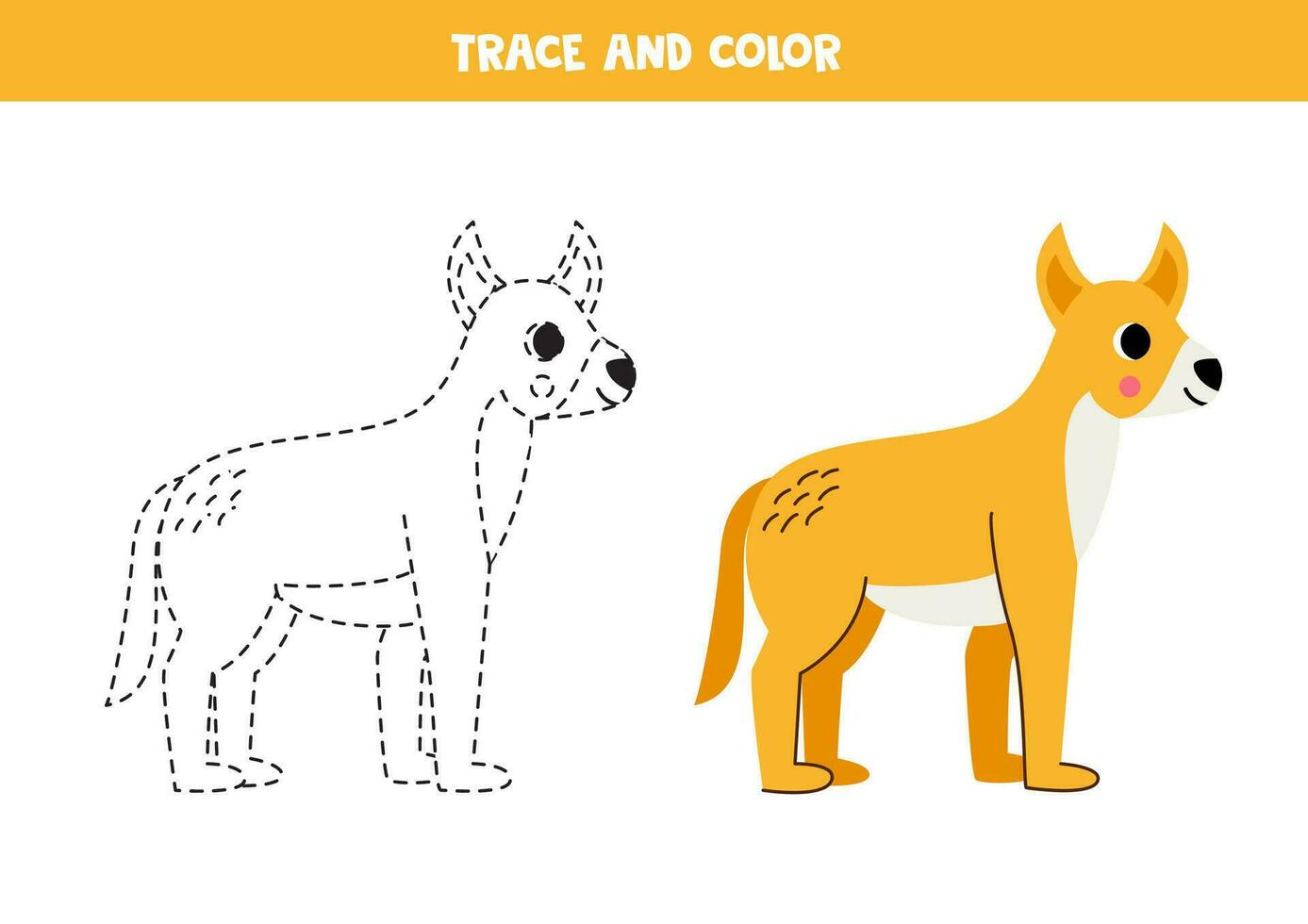This image, reminiscent of what you'd find in a children's coloring book or educational how-to guide, features a simple art instruction titled "Trace and Color." At the top, there's an orange bar stretching from left to right with bold white letters in all caps that read "TRACE AND COLOR." Beneath this header, against a plain white background, are two images of a dog, side by side. 

On the left, the dog is depicted as a stencil, outlined with black dotted lines. This side shows a simple sketch with pointed ears, a long tail, and a black nose. 

The right side displays the dog fully colored in. The dog is predominantly a warm yellow-orange color with brown-orange inner ears. It has distinctive white areas around its snout and belly, adding depth and highlighting its features. The dog's eyes, nose, and mouth are black, with a rosy-red cheek marked by a small circle. The areas along the inside of its front and back legs are outlined in black, providing subtle definition. This dual representation offers a clear, step-by-step example for children learning to trace and color.